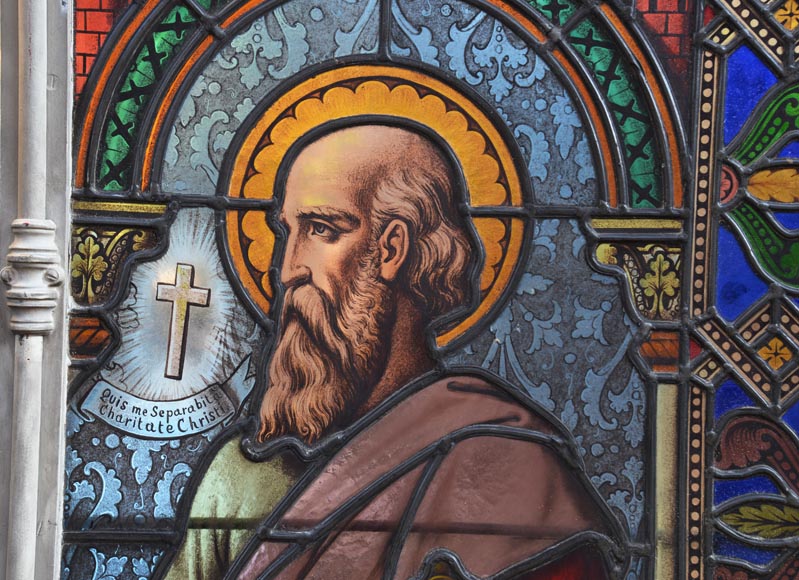This indoor photograph features a close-up of an ornate stained-glass window, vibrant in colors and meticulously detailed. Central to the window's design is the image of a saint, a white man with a bald head, and a long mustache and beard, donned in a brown and green robe, with a brown blanket draped over his green left shoulder. The man is depicted in profile, facing towards the left, with a serene composure.

The architectural design surrounding the saint includes an arched window frame, embellished with intricate patterns and vibrant hues. An orange circle acts as a halo behind the man's head, followed by a blue circle adorned with floral print designs. This is framed by the green arch itself, which is decorated with black X's and outlined by two orange borders. To the right of the arch, a decorative motif featuring elements in blue, red, orange, and yellow – resembling plant-like forms – adds to the window's ornate aesthetic.

On the left edge of the window stands a pillar, complementing the religious ambiance of the scene. A cross is prominently positioned in front of the man, shining brightly. Beneath the cross, in Latin script, are the words: "Quis me separabile charitate Christi," translating to "Who shall separate me from the love of Christ." The window's black outlines accentuate the detailed designs, enhancing the richness of the colors which include shades of green, orange, yellow, blue, red, cream, gold, and silver.